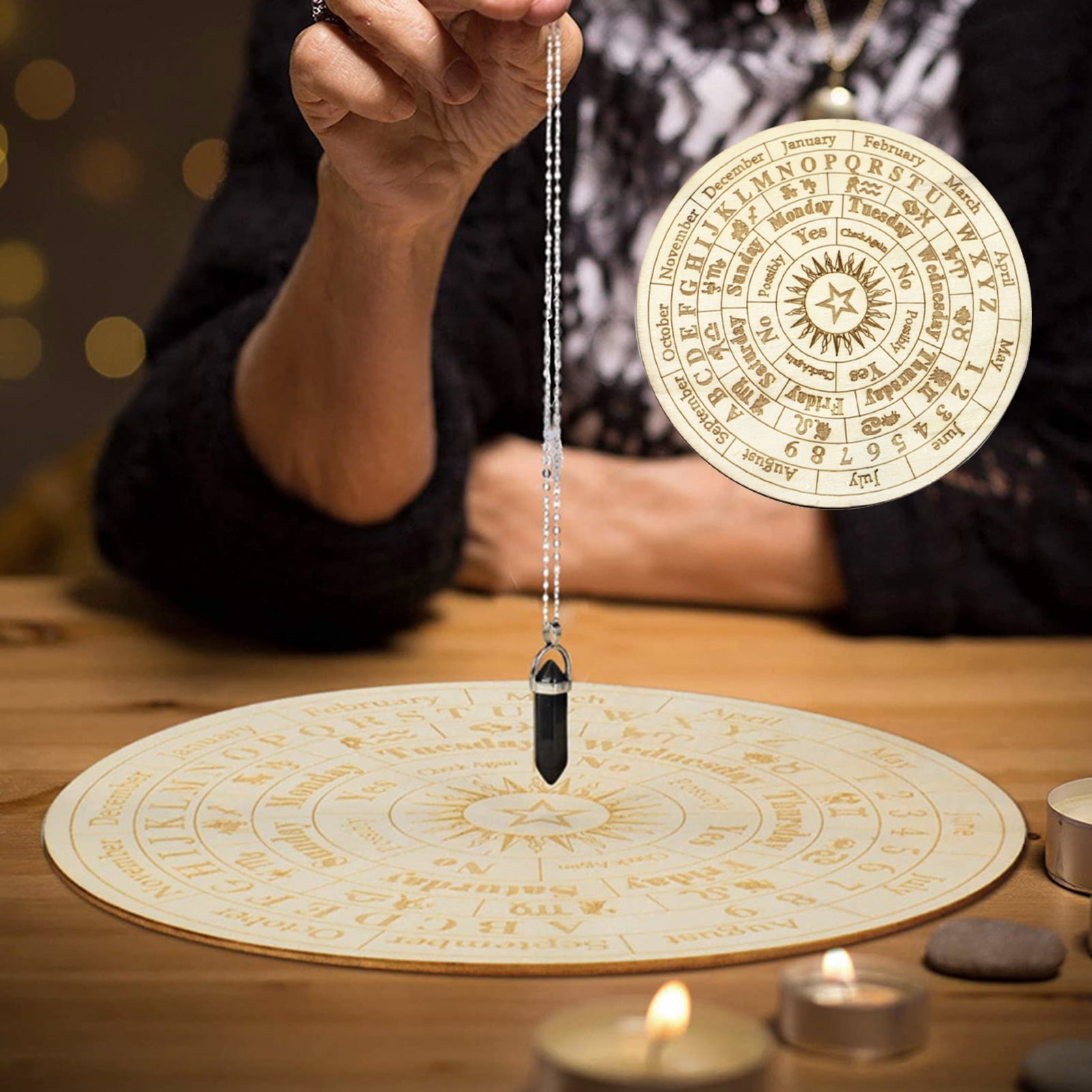The photograph portrays a mystical, New Age scene centered around an intriguing ritual. A person, whose face is not visible, is seated at a wooden table, holding a silver necklace with a black crystal pendant over a meticulously engraved round disc on the table. The disc features detailed inscriptions, including the months of the year, days of the week, letters, numbers, zodiac signs, and words such as "yes," "no," "possibly," and "check again," all arranged in concentric circles. A starburst design with radiant rays is prominently displayed at the center of the sun motif on the disc. The individual, wearing a black sweater with some white writing, clasps the pendant with their right hand, while their left arm is tucked underneath their right arm. Around the disc, there are small lit tea lights and stones enhancing the mystical setting. In the top right corner of the image, a close-up of the disc provides a clearer view of its intricate design. The overall impression is one of an astrological or witchcraft ritual, potentially an advertisement for the crystal pendant or the ritual platform itself.